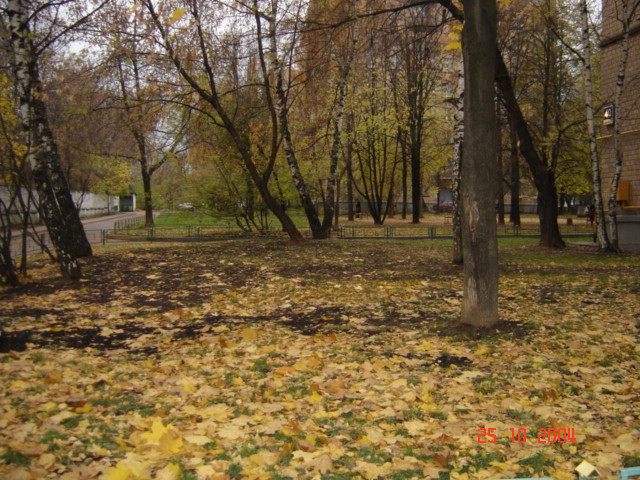The image, captured with a time stamp of 25-10-2004, shows a vivid autumn scene taken outdoors. The ground is predominantly covered in a beautiful mosaic of fallen leaves in shades of yellow and orange, though small patches of green grass poke through in certain areas. Tall trees surround the scene, with many of their branches now bare or sparsely adorned with remaining leaves in various autumnal hues. A driveway bordered by a metal fence and a road can be seen in the background, adding a structured element to the natural setting. To the right, a dark brown, slightly reddish brick house is partially visible, with a rusted-looking metal piece attached near its base, hinting at some utility function. Additionally, a man dressed in black can be seen walking towards the street in the distance. The overall setting, accentuated by the vibrant and scattered leaves, encapsulates the essence of a crisp fall day.